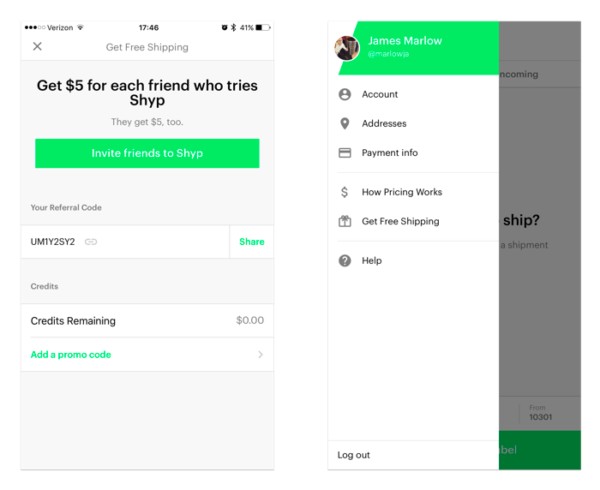This detailed screenshot displays two sections side by side.

**Left Section:**
- The top of the cell phone screen indicates a Verizon network and a Wi-Fi icon.
- The time reads 17:46, and there is a Bluetooth icon along with a 41% battery life indicator.
- Centered below the status bar is the prominent text "Get Free Shipping."
- To the left of this text is an 'X' icon for closing.
- In the next line, smaller text reads "Give $5 for each friend who tries SHYP (S-H-Y-P). They give $5 too."
- Below this line is a green rectangular button with the text "Invite Friends to Ship."
- Directly underneath is a gray section displaying the referral code "UMIY2SY2" with the option "Share" in green text to the right.
- Further down, a label reads "Credits Remaining: $0" followed by "Add a Promo Code" in green text at the bottom.
- The background of this section is predominantly gray.

**Right Section:**
- Appears to be part of a tab menu for a profile.
- At the top is the user’s name, "James Marlowe," against a green background with a profile picture to the left.
- Below the name, the menu options are listed as "Account," "Addresses," "Payment Info."
- A horizontal line separates this section from the next set of options: "How Pricing Works," "Get Free Shipping," and "Help."
- At the bottom of this list is the "Logout" option.
- The background here is a holographic gray, with the bottom part of this section also featuring green elements. 

The entire layout suggests an app interface designed for inviting friends, managing user profiles, and accessing various features and settings.